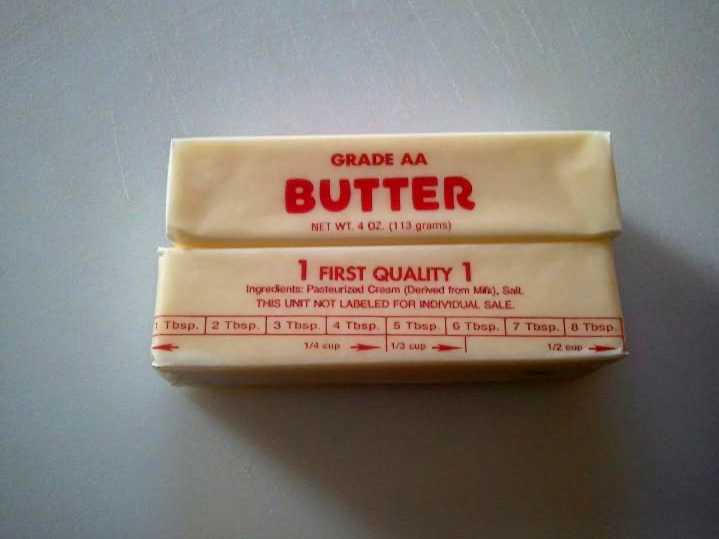This close-up photograph captures two sticks of butter lying on a pale gray, subtly scratched surface. The top stick of butter is oriented horizontally, with its wrapper displaying "Grade A Butter" prominently in red print, followed by the weight designation "Net Weight, Four Ounces." The second stick of butter beneath it is turned to reveal a different side of its packaging. This stick features the text "First Quality" in red print, which is followed by the listed ingredients: "Pasteurized Cream (derived from milk), Salt." Additionally, it bears the notice "This unit is not labeled for individual sale." The wrapper also displays precise measurement markings, including increments for one tablespoon, two tablespoons, three tablespoons, and so on, as well as measurements indicating a quarter cup, a third of a cup, and a half cup, which aid in culinary applications.